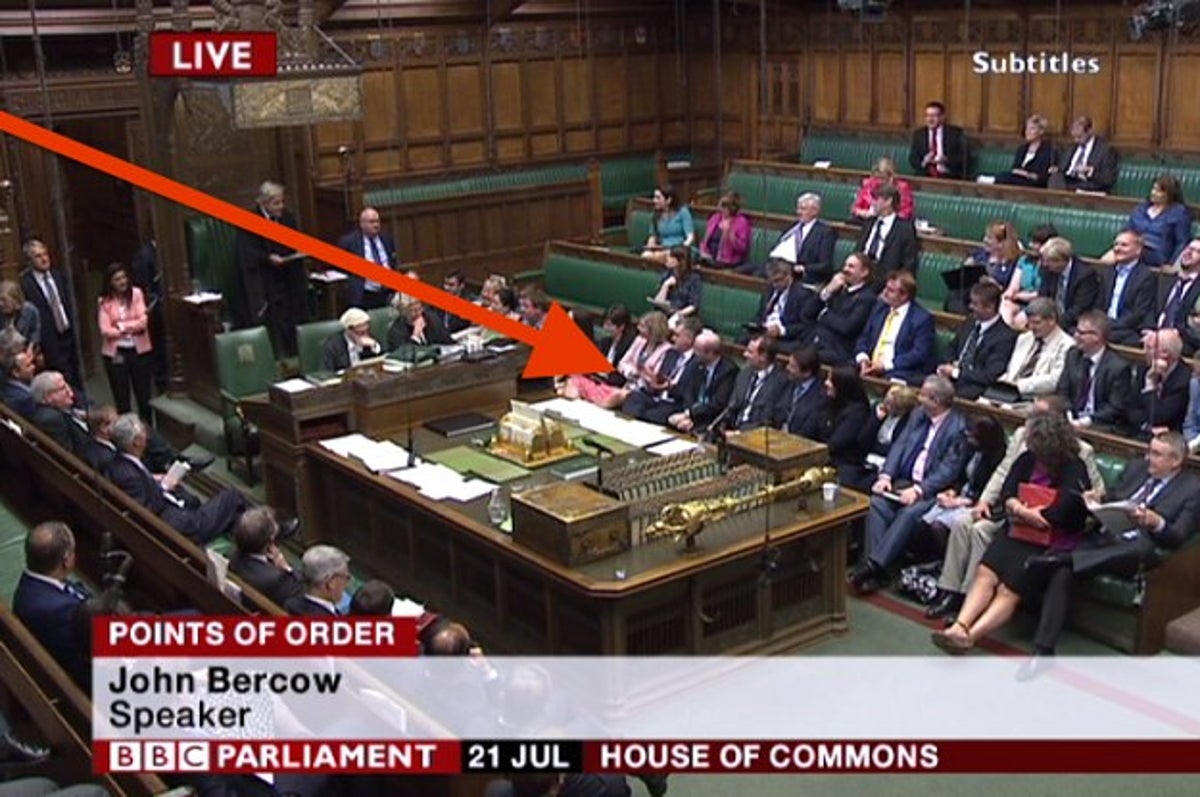This image is a detailed screenshot from a live broadcast of the proceedings in the House of Commons in Britain on July 21st, aired by BBC Parliament. The bottom of the screen displays captions reading, "points of order, John Bercow speaker" with an additional text, "21 July, House of Commons." An orange arrow originating from the top left corner points to a specific woman seated in the first row, who is dressed in a white blazer and pink pants. She is attentively looking towards a judge positioned in the top left corner, elevated on a green high chair. The judge is accompanied by a bailiff in a black suit situated to his left, and two individuals occupying chairs directly beneath him. The image also features rows of people in suits and dresses, indicating a formal setting akin to a courtroom or meeting room. In the top right corner, there is a "Subtitles" label in white text and a "Live" indicator on the left side, confirming the live nature of the broadcast. The scene includes a central table adorned with a scale model of a building surrounded by model grass, further emphasizing the structured and official atmosphere of the setting.